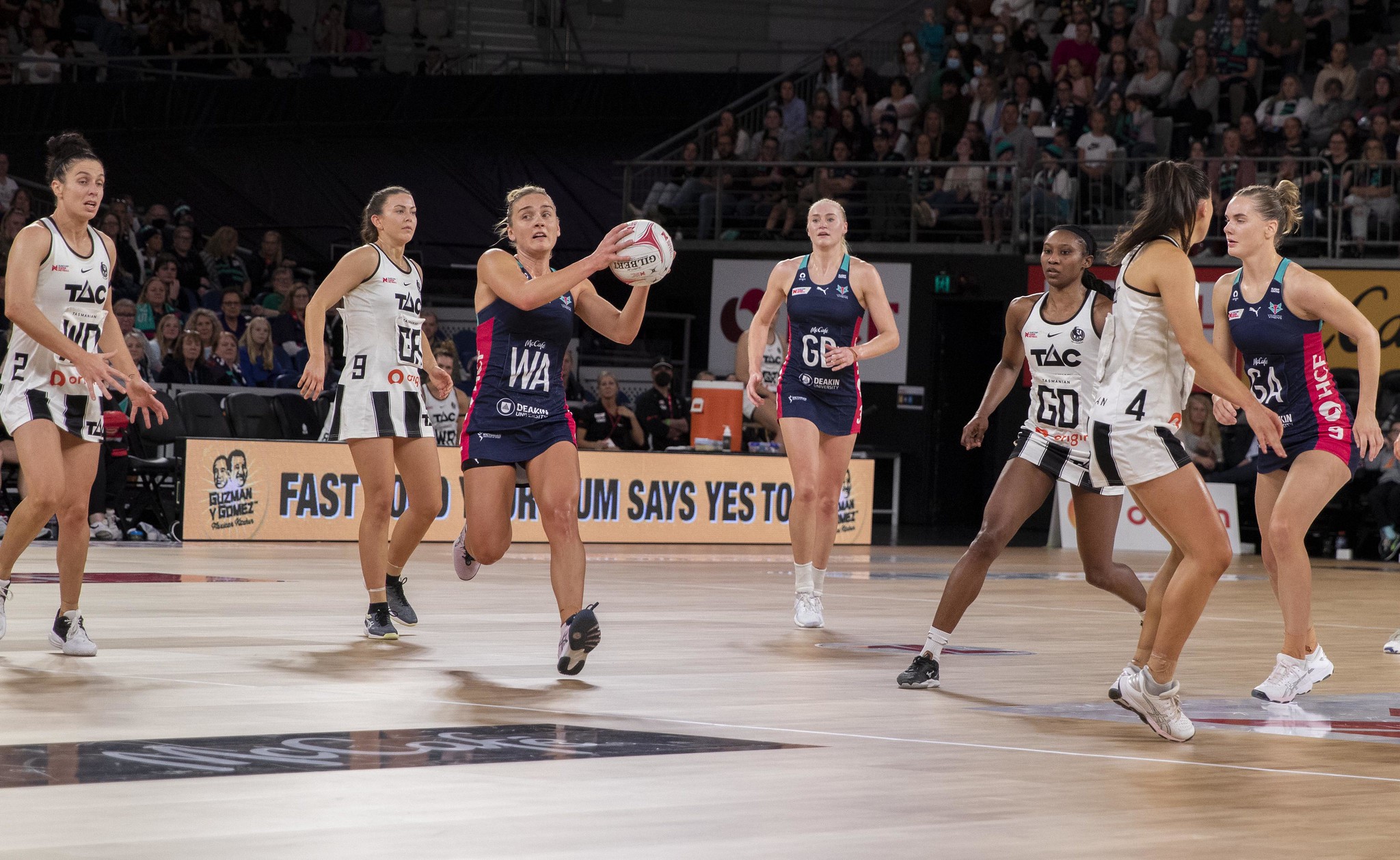This is a detailed photograph capturing an intense moment in a women's basketball game. At the center of the image is a woman clad in a black and black jersey with white lines running down both sides and a prominent "WA" on the front. She is holding a white basketball adorned with a red line pattern. Surrounding her are seven other players: three teammates in matching black jerseys with white and red accents and four opponents wearing white tank tops and black and white striped shorts. The action appears to be moving towards the camera, giving a dynamic, in-the-moment feel to the image.

Behind the players, the photograph shows a busy spectator area filled with people watching the game. The gymnasium floor is wooden, typical of indoor sports arenas. On the right side of the image, there is a glimpse of a table with a large Gatorade container, suggesting the presence of judges or coaches closely monitoring the game. Despite the lively activity in the foreground, various signs in the background are partially obscured by the crowd, adding to the sense of a bustling and engaging competitive environment.